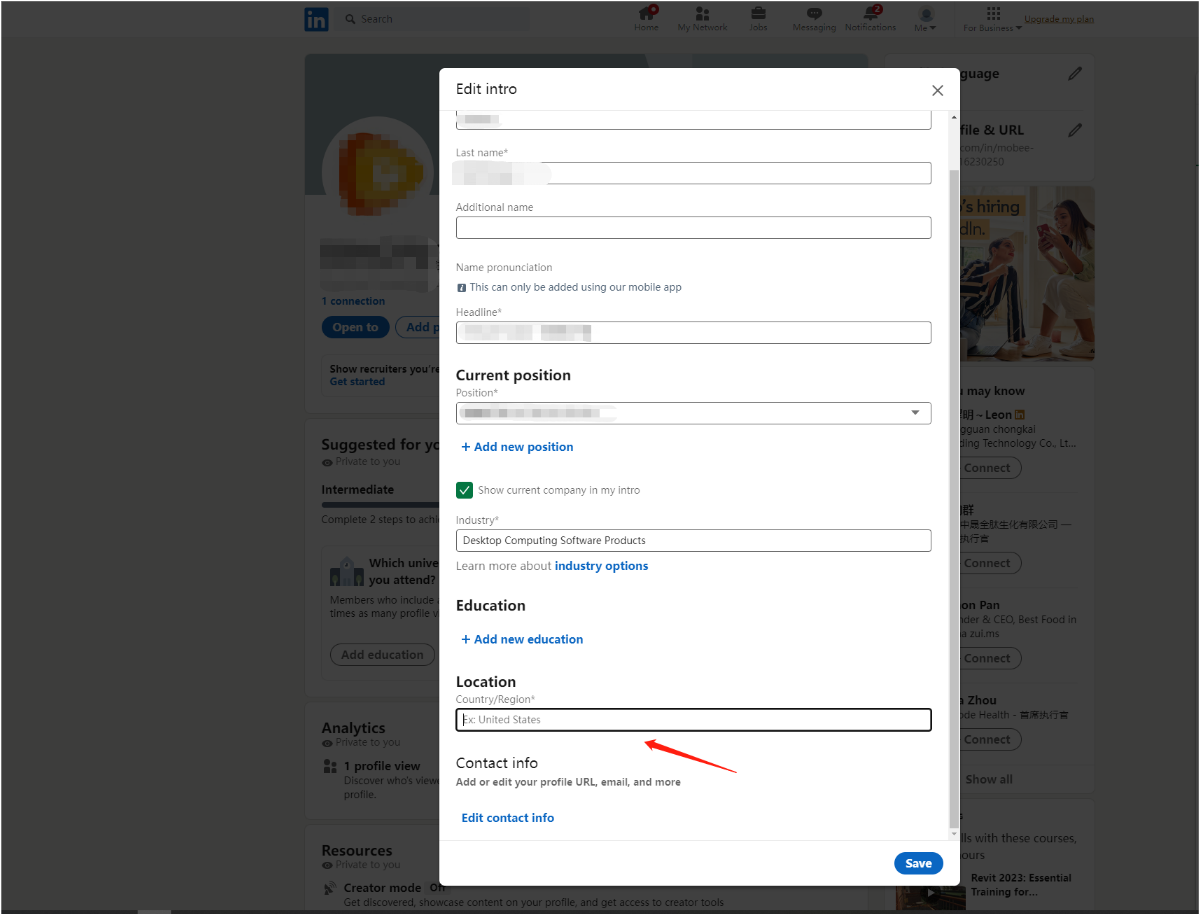The image depicts a somewhat wider-than-tall interface of a LinkedIn page, characterized by a semi-transparent overlay reminiscent of a grayed-out window background. At the top, the recognizable LinkedIn logo is situated approximately a quarter into the grayed-out area, flanked to the right by a prominent search bar and several navigation buttons, their legibility obscured by the overlay.

Beneath the header, the left sidebar houses a series of navigation boxes labeled "Suggested for you," "Analytics," "Resources," and more, indicating various site features. On the right-hand side, the interface showcases a list of potential connections, identifiable by multiple "Connect" buttons, approximately four in total, which occupy about 40% down the page. Above these, a graphic illustration portrays a man engaged in conversation with a woman looking to the left.

Dominating the center is the main window of interest, a rectangle roughly twice as tall as it is wide. It is labeled "Edit Intro" at the top and includes a sequence of editable fields for "First Name," "Last Name," and "Additional Name," suggesting that this section allows users to modify their LinkedIn profile information.